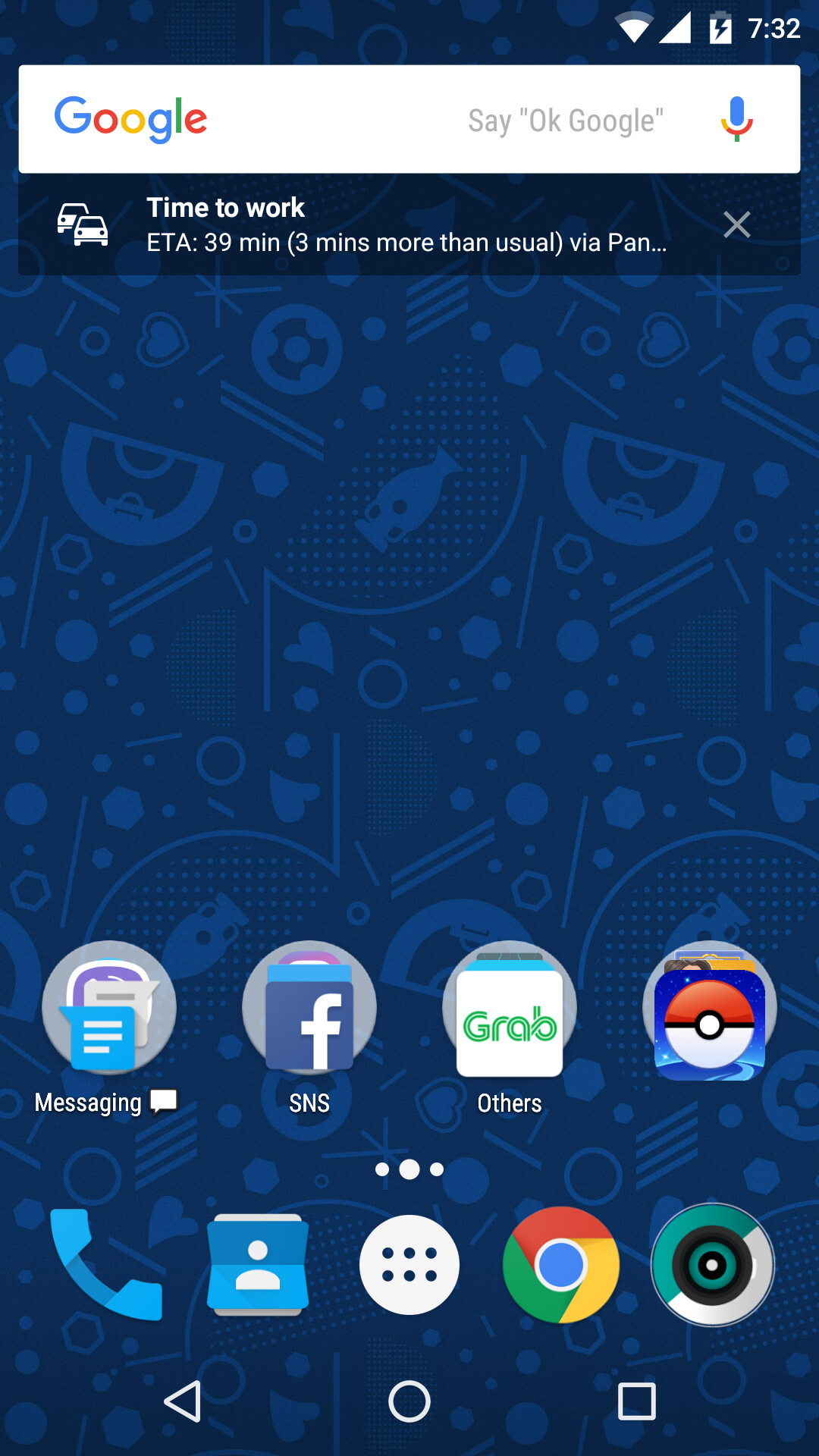Screenshot of a smartphone home screen displaying various elements against a blue background. At the top, a search bar with the Google logo and a microphone icon is visible, accompanied by the text "OK Google." Below this, a notification reads, "Time to work; ETA: 39 minutes (3 minutes more than usual) via PAN..." with an 'X' for dismissal. The status bar shows the time as 7:32, along with other standard icons such as battery life and signal strength.

Several app icons are prominently displayed, including Messaging, SNS, Phone, Contacts, a Google Chrome symbol, and a camera icon resembling a camera lens. Additionally, there is a white circle consisting of two rows of three blue circles each, suggesting some form of a menu or app drawer. At the bottom, the navigation bar presents three functional icons: an arrow pointing to the left (Back), a circle (Home), and a square (Recent Apps).